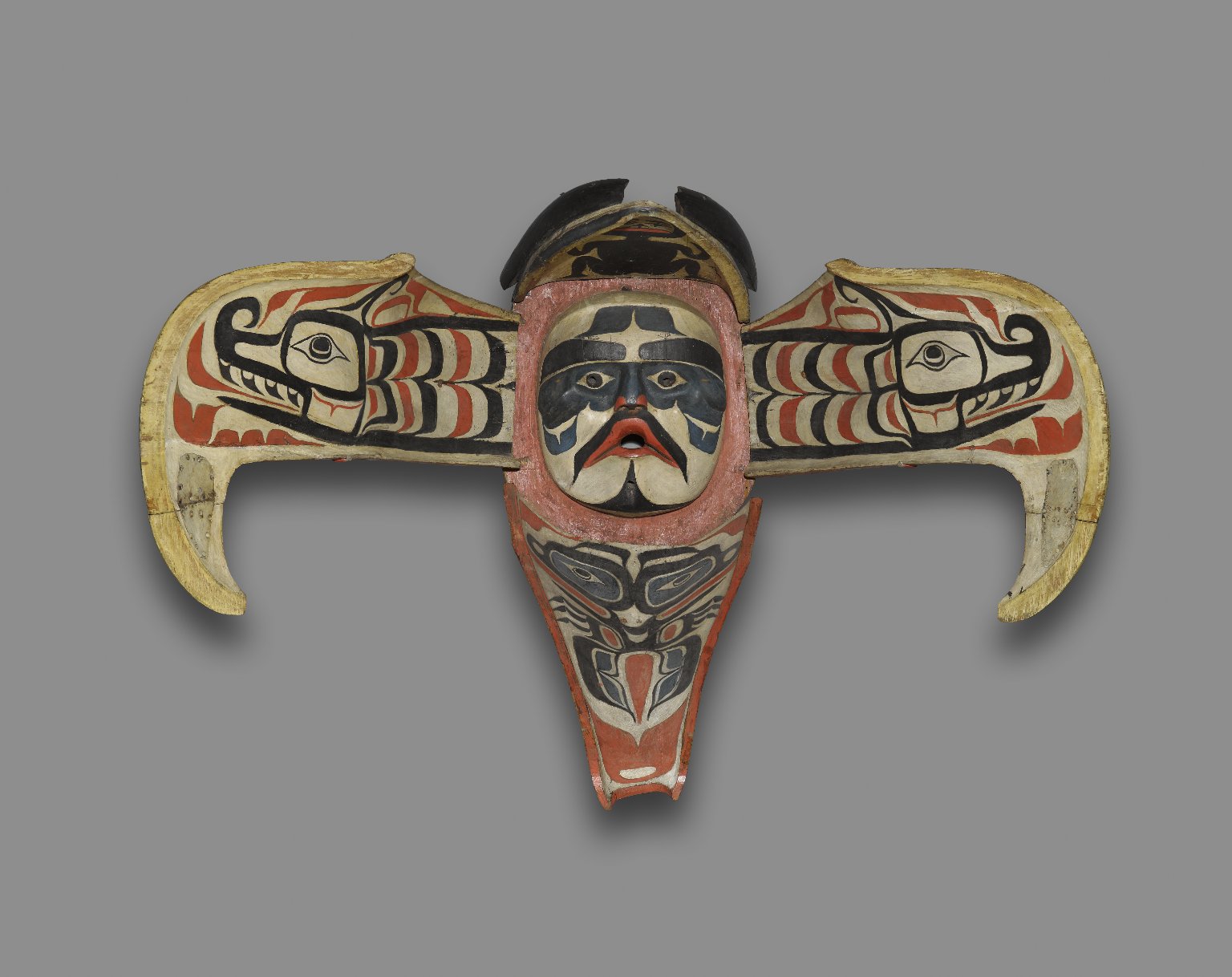This color photograph showcases a meticulously detailed indigenous American wood carving, reminiscent of a totem pole. At the center of the composition is a prominently featured human face, accentuated by its white complexion and adorned with intricate black decorative paint. The face is further highlighted by its vivid red lips and slightly open mouth. This central face is set against a rich red backdrop, and a distinctive visor-like element arches over it.

Emerging from both sides of the central face are elaborately carved and painted wings. These wings feature striking imagery of black and red serpentine figures with pronounced teeth and curved black noses, set against a white background. The wings elegantly curve downward, bordered by a shimmering gold trim along their outer edges.

Additional elements include a secondary human figure situated on the visor-like extension. This figure is depicted in black against a white background, further contributing to the intricate and layered design. Below the central face, the carving extends into a neck-like structure painted in hues of red and blue.

Surrounding the entire carving is a gray background, which contrasts with the vibrant colors and intricate details of the artwork, further emphasizing its craftsmanship and cultural significance.